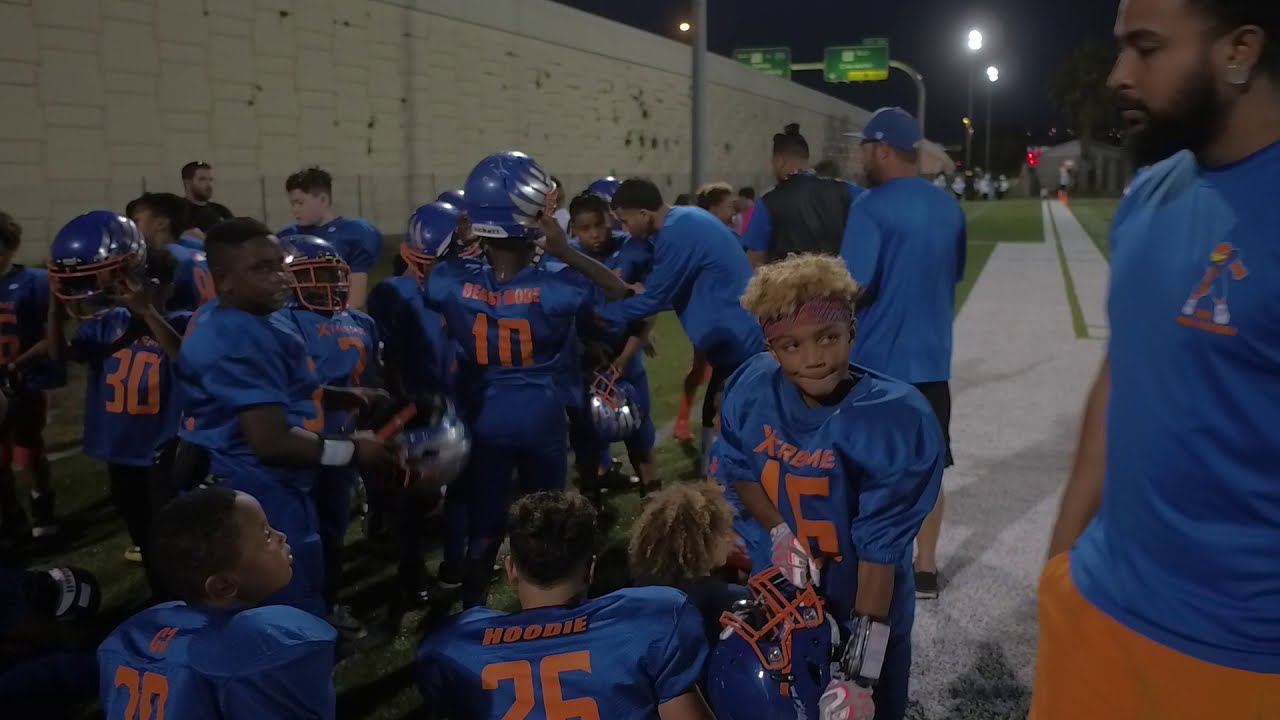This image captures a group of youth football players and a couple of their coaches, possibly with some parents nearby, gathered along the side of a busy highway, distinguished by green informational signs and a "Exit Only" indicator. The setting features a light gray sidewalk with green grass on either side, leading towards additional people in white uniforms, suggesting another team. The team consists predominantly of African-American boys, with a few visible Hispanic and Caucasian players, all in blue jerseys adorned with orange numbers and the word "Xtreme" on the front. Their helmets are also blue, accentuated with silver streaks. Some players are seen either putting on or holding their helmets, while others have them already on. 

One coach, an African-American man with a beard, stands out in his blue shirt marked with an orange team logo, paired with bright orange pants. Specific details are visible on the players' uniforms: for instance, one boy facing the camera wears jersey number 16 and holds his helmet, wearing a distinctive gray, pink, and white glove. Another player's back showcases the name "Beast Mode" with the number 10, while "Hoodie" and the number 26 appears on another. The numbers 30 and 20 are also visible among the players. The bustling city environment and signs of passerby cars emphasize the vibrant urban setting adjacent to where the team momentarily congregates, likely either before or after their game.